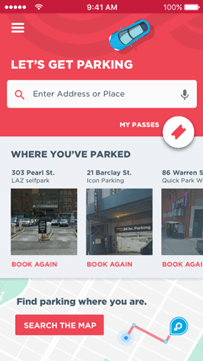Screenshot of a Mobile Parking Application:

The image is a screenshot of a mobile parking application interface. At the very top, the status bar displays various icons including the cell phone signal strength represented by five circles, the Wi-Fi symbol, the current time (9:41 a.m.), and the battery indicator showing 100% charge.

Just below the status bar, a navigation hamburger button is situated in the top-left corner. Adjacent to this, a blue car icon is set against a red background. Beneath this header, the text "Let's get parking" is displayed above a search bar, which prompts the user to "Enter address or place." The search bar features a magnifying glass icon on the left side for text searches and a microphone icon on the right side for voice searches.

Below the search bar, the section labeled "My Passes" contains a white circle with a logo resembling a ticket stall. Underneath, the bold text "Where You've Parked" introduces three saved parking locations. Each location entry includes an address, an image of the respective parking lot, and the option to "Book Again."

Further down, a map image is visible with the caption "Find Parking Where You Are." This section encourages users to locate nearby parking spots and features a red button labeled "Search the Map."

Overall, the mobile application's screenshot provides a detailed and organized layout for users to search, save, and manage their parking spots efficiently.